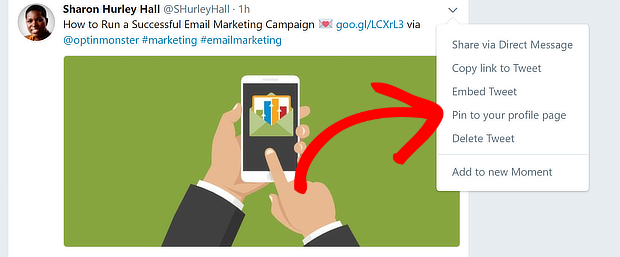In this screenshot of a social media post made one hour ago on Twitter by user Sharon Hurley-Hall (@shurleyhall), a comprehensive guide on running a successful email marketing campaign is being shared. The post features a shortened URL (goo.gl/lcxrl3) that directs followers to the detailed content, shared via the marketing platform OptinMonster. The hashtags #marketing and #emailmarketing are used to categorize the tweet for broader reach within those communities.

Dominating the center of the screenshot is an image depicting a hand holding a mobile device and tapping on the screen. A red arrow extends from the hand's right index finger to highlight the option "Pin to your profile page," providing visual guidance on how to pin the tweet for easy access on one's Twitter profile.

Surrounding this main image are various Twitter interface options, including "Share via direct message," "Copy link to Tweet," "Tweet," "Embed Tweet," "Pin to your profile page," "Delete Tweet," and "Add to new Moments," giving a comprehensive overview of actions that can be taken with the tweet.